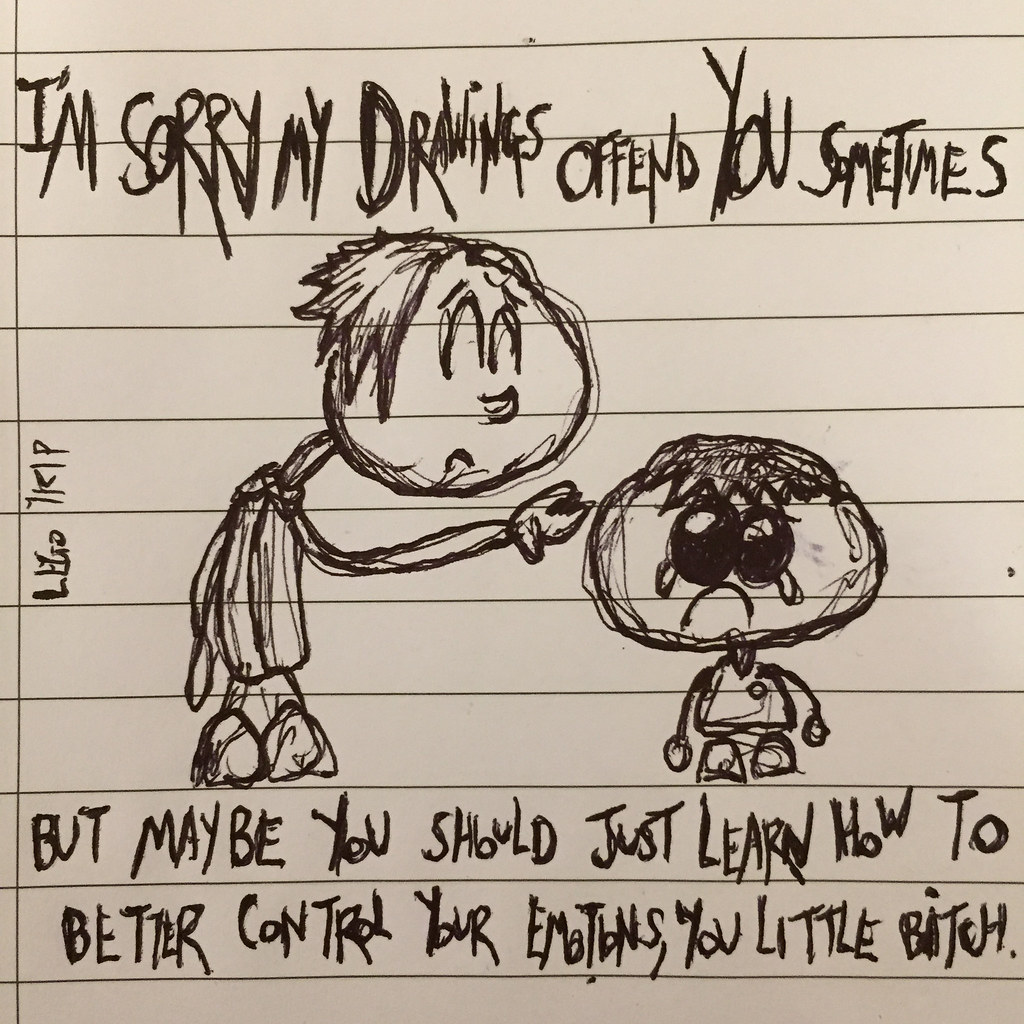The image is a square-shaped photograph of a pencil and ink drawing on light-colored, lined notebook paper. The paper features horizontal dark lines. At the top of the drawing, in scratchy, hand-drawn black lettering, it says, "I'm sorry, my drawings offend you sometimes." Below this, there is a crude, stick-figure-like illustration. On the left side, there is a taller figure with a circular head sporting a small patch of hair. The figure has simplistic facial features, including upside-down U-shaped eyes with dashes above them for eyebrows, a small mouth, and an inverted U for a chin. The left figure extends one arm towards a shorter figure on the right, who appears to be crying. This smaller figure also has a circular head, dark eyes with tears, and a small, circular body with stick arms and legs. The smaller figure looks younger and is visibly upset. At the bottom of the drawing, more scratchy text reads, "but maybe you should just learn how to better control your emotions, you little bitch." To the left of the drawing, there might be an indistinct signature and date, adding a possible context of being drawn by a student.